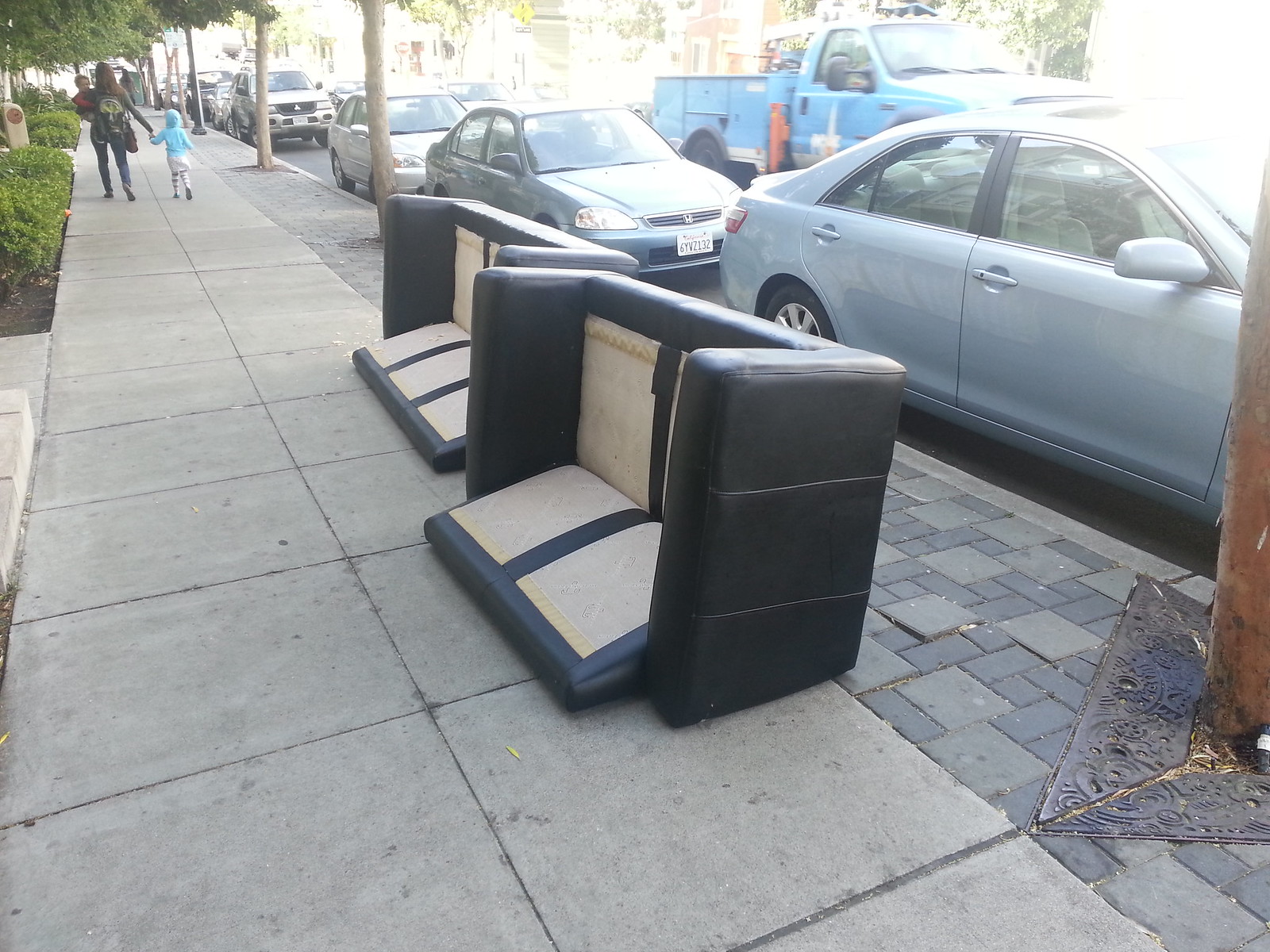The image captures a busy city street with a long gray sidewalk in the foreground. Along the curb, a row of gray and blue cars is parked, including a blue utility truck. Prominently featured on the sidewalk are two identical black couches, tipped onto their backs. The seats are missing their cushions, exposing a contrasting cream or white interior. The couches, seemingly in good condition, may be in the process of being moved. At the far end of the sidewalk, a woman dressed in a black shirt and blue jeans walks away, holding a small child and the hand of a little girl in a blue hoodie, white skirt, and black and white socks. Behind them and above their heads, green trees and shrubs line the street. Power lines crisscross above, completing the urban scene.